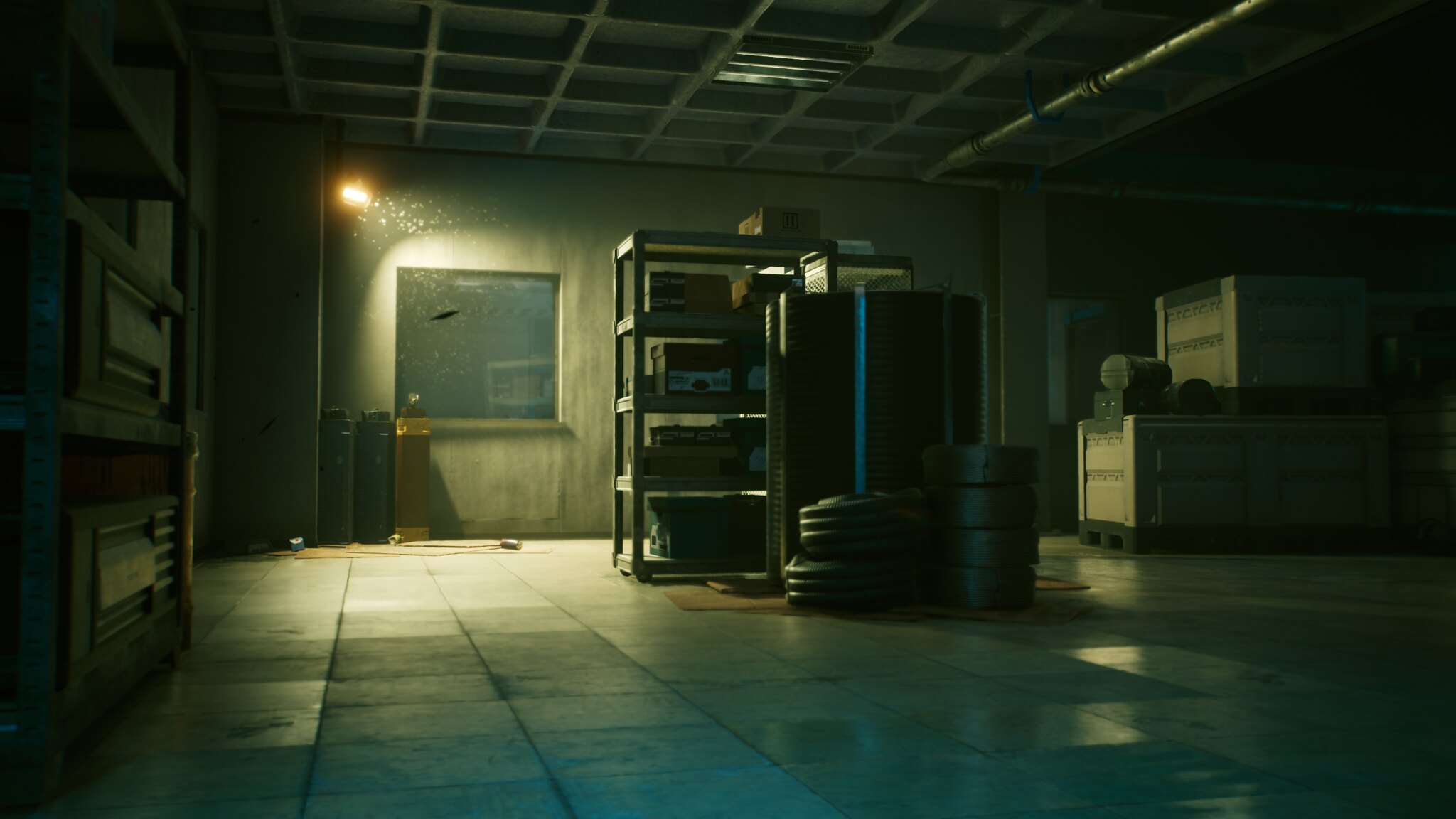The image presents a dimly lit, warehouse-like room that appears to be a blend of reality and a 3D environment, potentially for a video game. The floor is covered with square tiles, possibly in shades of light green, blue, or gray, which reflect light in certain areas. Central to the room is an industrial metal shelf filled with several black or cardboard boxes, devoid of visible labels. In front of the shelf, a neat stack of tires sits on the floor. The room also features a metal crate and a smaller one on top of it, located to the right side of the image. The walls are largely unadorned but include a bright light source mounted above a hazy square window on the center-left, emphasizing the room's sparse, industrial character. The ceiling is patterned with square units and contains visible metal pipes. The overall scene is barren yet meticulously organized, suggesting a utilitarian purpose for the space.